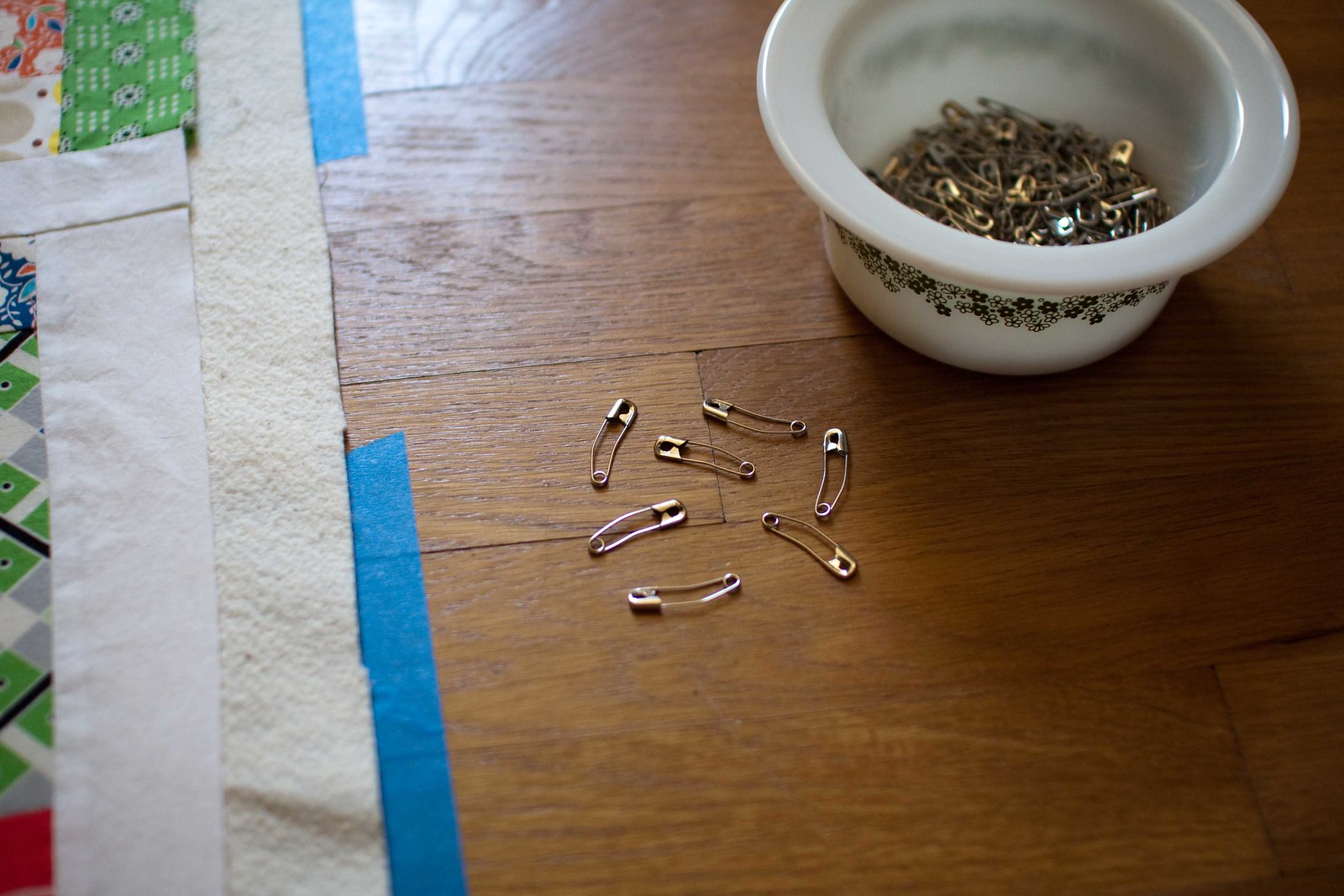The photograph captures a scene on a hardwood floor characterized by rich brown and tan hues. To the left of the frame, partially obscured, lies a cloth or paper towel with a colorful pattern, suggesting it could be part of the artistic setup. Central to the image are several small safety pins, arranged in a neat, closed position. These safety pins, in silver and gold hues, seem purposefully placed on the floor, perhaps indicating their use in an ongoing craft project. 

To the upper right of these pins is a white ceramic bowl with a delicate black floral pattern around its base. This bowl is filled with more safety pins, matching those on the floor in both size and color. The careful composition of the elements—safety pins both inside and outside the bowl, the patterned cloth, and the distinct hardwood floor—hints at an artistic process rather than a product display. The natural light casts a shadow from the bowl, enhancing the textured wood grain and adding depth to this intriguing, craft-centered snapshot.